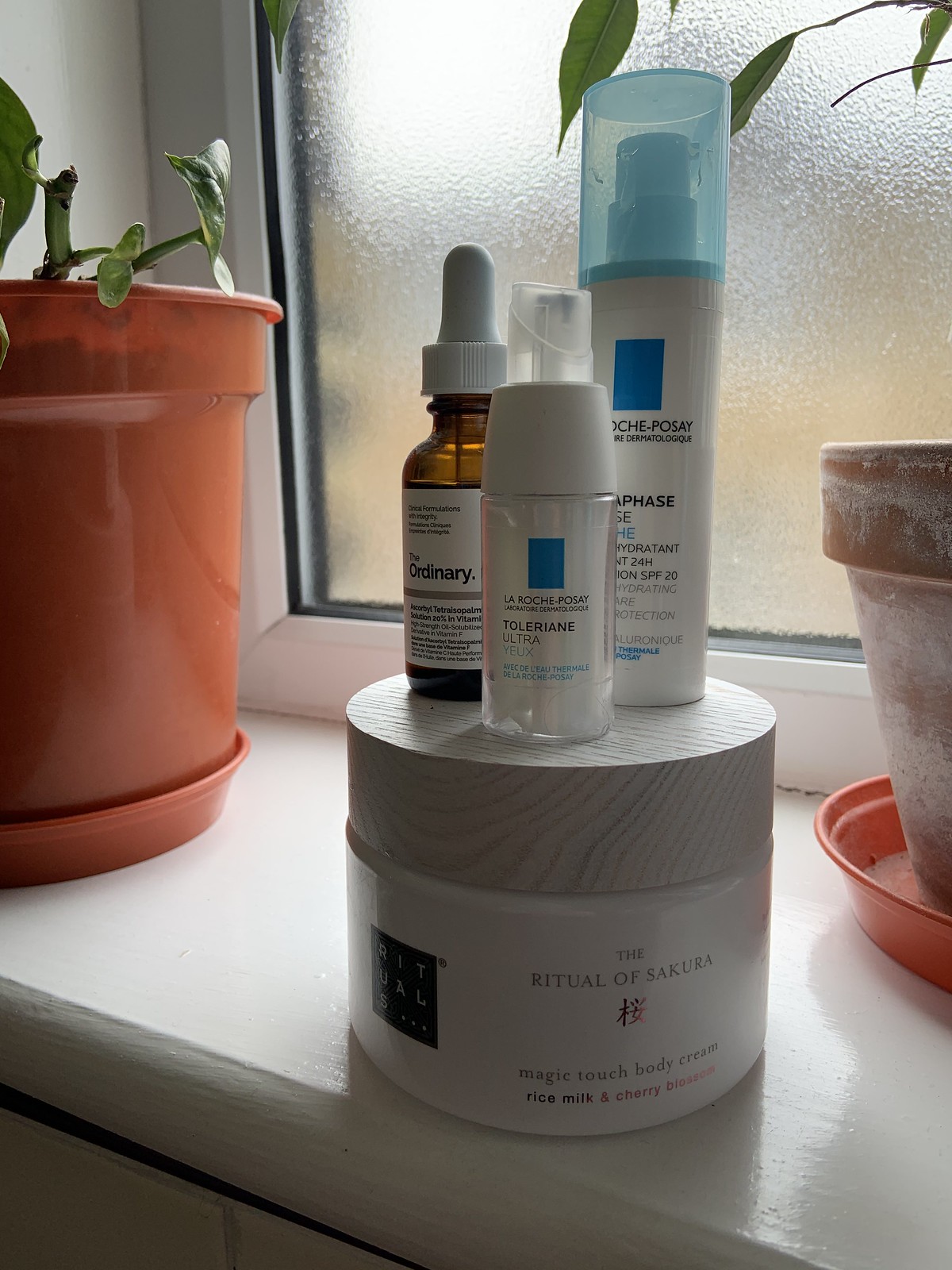A windowsill scene bathed in soft, diffused light from a frosted window, characteristic of a bathroom setting. The windowsill hosts an array of beauty products, including a white canister of "The Ritual of Sakura" body cream, exuding an inviting cherry blossom scent. Adjacent to it, three bottles stand in a neat row: the first, a dropper bottle from The Ordinary, and the other two featuring a blue square logo with indistinct writing. The arrangement is flanked by two distinct pots—the one on the left, a terracotta-colored plastic pot, displays sprouting green buds, while the right holds a white pot without any visible plants, sitting atop a matching terracotta-colored dish designed to catch excess water.